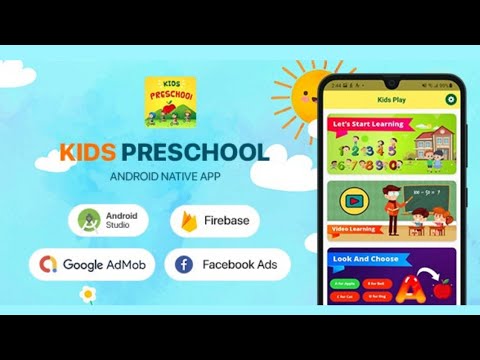The image appears to be a partial screenshot of a preschool website, likely captured from a tablet or laptop. The screenshot shows visible borders at the top and bottom of the image, which are both black and of the same height, but no side borders can be seen. 

At the center of the image, slightly skewed to the left, the text "Kids Preschool" is prominently displayed. The word "Kids" is highlighted in an orangish-yellow font, while "Preschool" is rendered in a bluish color. 

Above this central text, "Kids Preschool" appears again, this time within a hand-drawn media image that resembles a book, suggesting it’s an application or a resource for children. 

Directly below the main "Kids Preschool" text, the words "Android Native App" are visible. Below this, aligned slightly to the left, are the phrases "Android Studio," "Firebase," "Google AdMob," and "Facebook Ads," each accompanied by their respective icons.

The background of the image features a partially visible sun with some clouds against a sky. Additionally, there is an image of a phone, displaying various educational images for children, including numbers and letters, reinforcing the preschool theme.